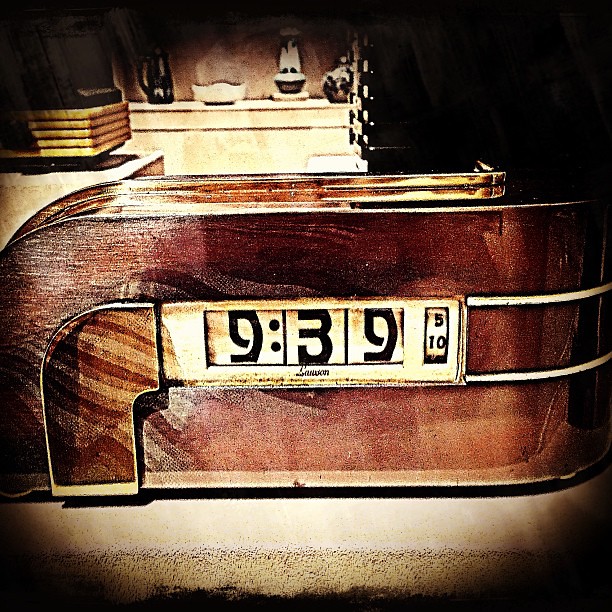This image features a uniquely designed wooden clock with an artistic, wave-like shape. The clock face is carved from rich, dark wood, with a rectangular form that has a rounded top left corner. This design creates a dynamic wave effect that starts from the bottom left and sweeps gently upward before curving to the right. At the center of the clock is a white digital display reading "9:39:10," capturing a precise moment in time. The craftsmanship of the wooden frame contrasts beautifully with the modern, minimalist digital display, blending traditional materials with contemporary design.